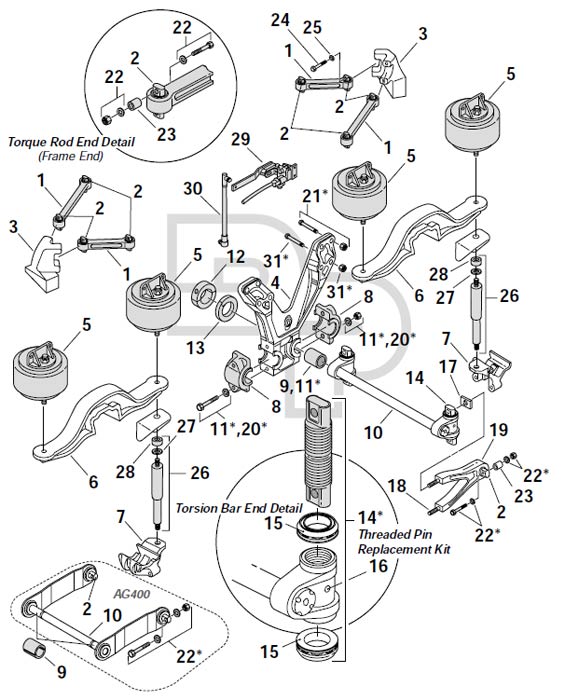The image is a highly detailed and intricate schematic mechanical drawing, primarily in black and white with touches of gray, showcasing the steps to assemble a torque rod and torsion bar. The diagram presents an exploded view of numerous small, intricately illustrated parts, each meticulously labeled and numbered in succession from 1 to 31, detailing the sequential steps. Key areas in the drawing include labeled sections such as "Torque Rod End Detail" and "Frame End" in the top left, "Torsion Bar in Detail" and its components in the bottom middle, along with "Threaded Pin Replacement Kit" in the bottom right. Despite the comprehensive numbering and labeling with arrows pointing to specific parts, the arrangement can appear somewhat chaotic, making it challenging to visualize the fully assembled outcome. Additionally, a watermark "DP" is subtly present in the background. This illustration, while dense with information, serves as an extensive guide for the assembly process, likely related to car suspension components.